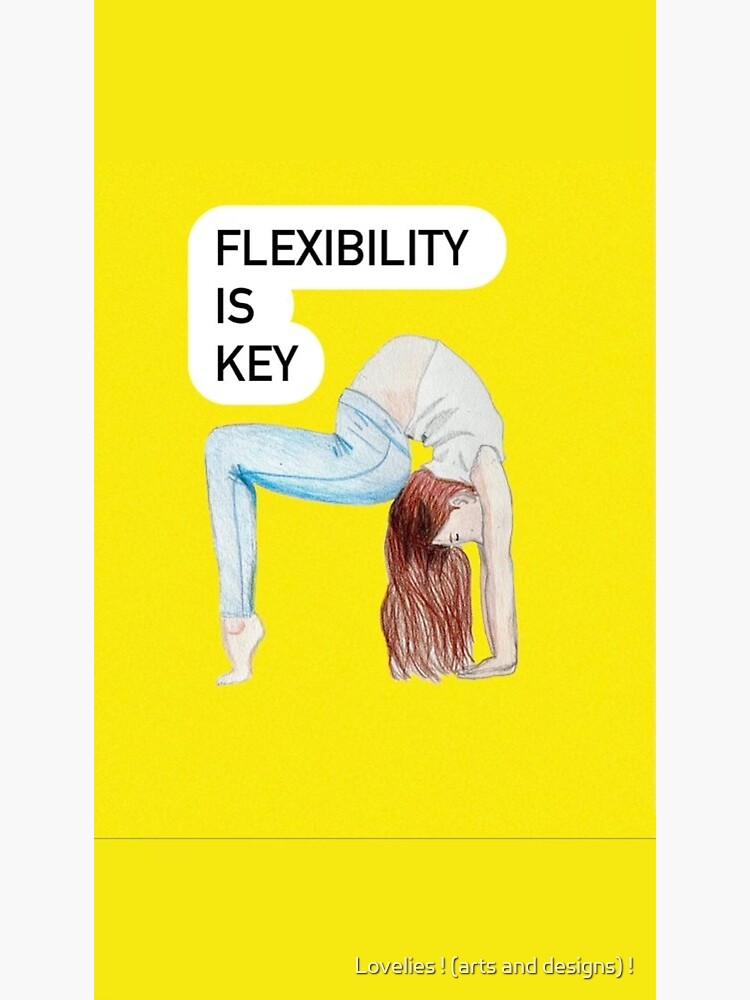The image features a vertical illustration with a vibrant yellow background, bordered by vertical pink lines on either side. The primary focus is a detailed, colored pencil drawing of a brown-haired woman performing an impressive flexibility pose. She is bending backwards so dramatically that her back arches at two 90-degree angles, resulting in her arms being parallel to her legs and her hair hanging vertically in line with gravity. Her pose gives the impression of standing on her tippy toes with her hands flat on the floor, showcasing remarkable flexibility. At the top of the image, centered in bold black text encased in white bubbles, is the motivating phrase "Flexibility is Key," with each word on a separate line. Additionally, at the bottom of the illustration, there is a small white text with a black drop shadow that reads "lovelies! (arts and designs)!" for a finishing touch. She is depicted as wearing jeans, adding a touch of casual realism to the stylized artwork.